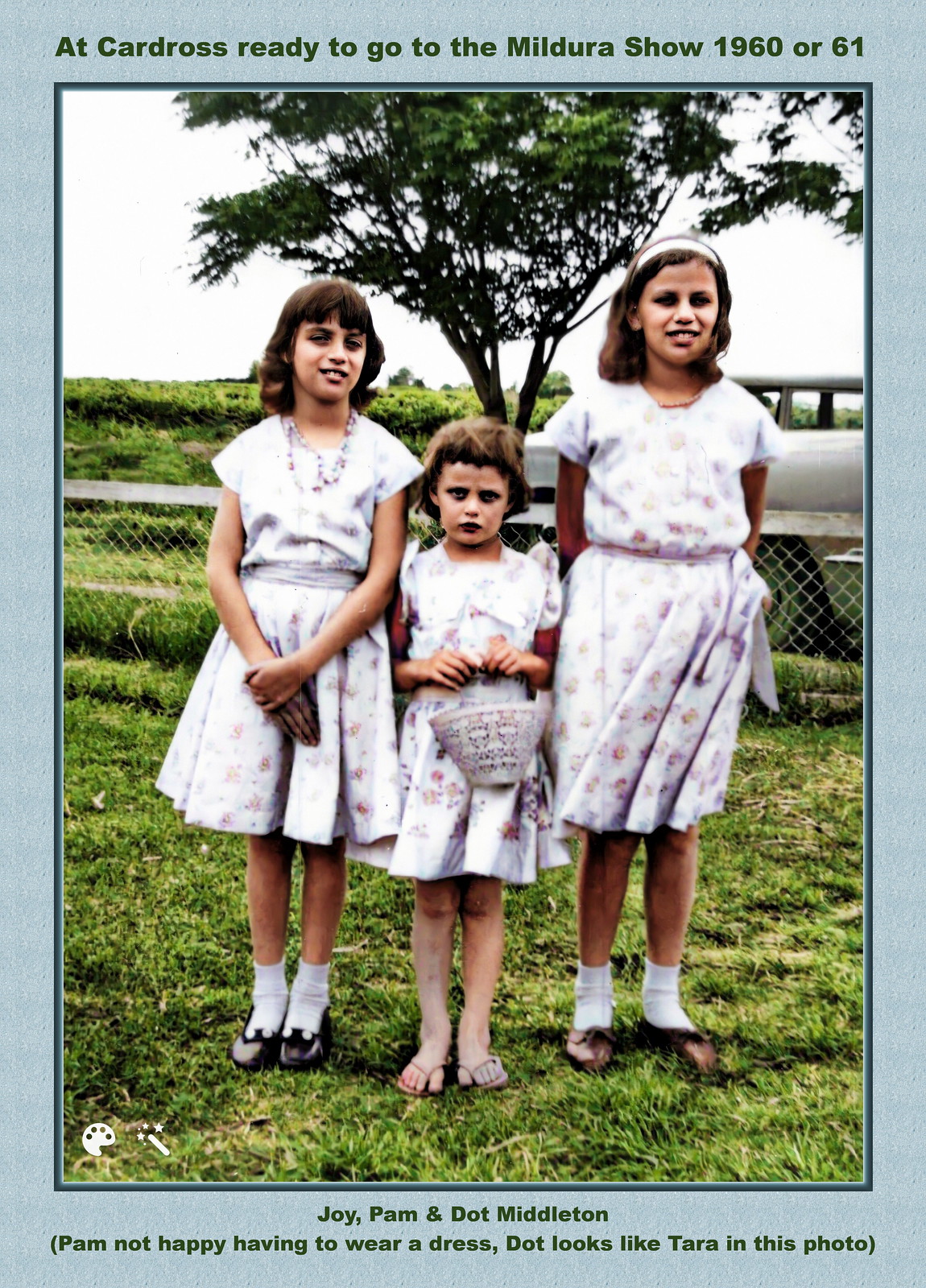In this nostalgic photograph from 1960 or 1961, taken at Cardross, three young sisters—Joy, Pam, and Dot Middleton—stand on a grassy field, ready to attend the Mildura show. The girls, dressed in pretty floral dresses, are of varying heights with Joy being the oldest, Pam likely unhappy about wearing a dress, and Dot resembling another family member named Tara. Above them, a green caption reads, "At Cardross ready to go to the Mildura show 1960 or 61." Below the photo, another caption lists their names, reiterating Pam's discomfort and Dot's resemblance to Tara. The image is set against a backdrop featuring a chain-link fence, a partially visible white car, and a tree with a distinctive Y-shaped trunk. The lighting casts an unusual shadow around the girls' eyes, adding an unintended sinister effect to this evocative family snapshot.